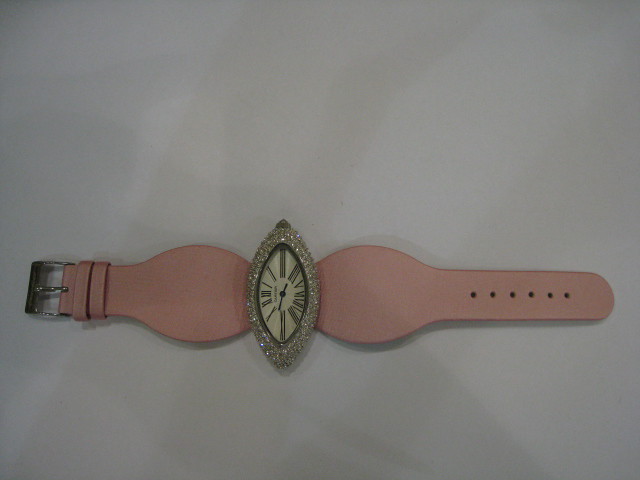This wristwatch is a strikingly unusual timepiece with a distinctive design. The band is crafted from leather and features a unique dusty mauve color. Unlike typical straps, this one maintains a standard width until it nears the watch face, where it interestingly bulges out. The clock face itself is an unconventional shape, similar to an elongated oval but with pointed ends. It is an analog watch, exuding a vintage charm with its ivory-colored interior. The hour and minute hands, set against black numbers, are striking despite the numbers being artistically stretched and distorted. Adding to its ornate design, the watch’s crown is encircled with tiny, sparkling stones, which appear to be either diamonds or rhinestones. The clasp shows signs of significant wear, indicating its age and extensive use. Overall, this unique watch combines aged elegance with distinctive style elements.